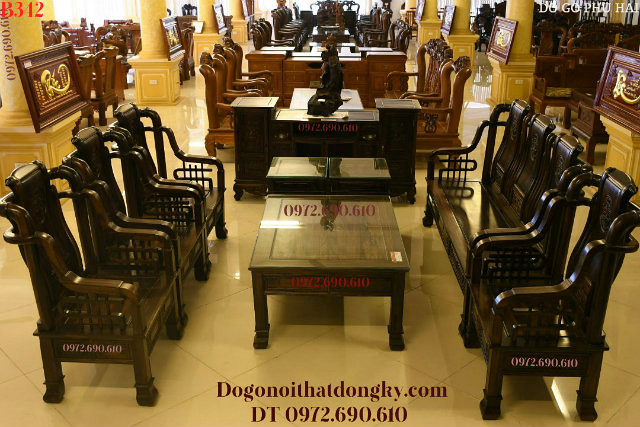This image depicts a furniture store showcasing various wooden tables, chairs, and benches. The foreground features a dark brown wooden table with a glass top, surrounded by matching dark brown chairs. Adjacent to this setup is a wooden desk. Behind these, a similar arrangement of light wood furniture, including chairs, tables, and a desk, is displayed. The store's marble floor with distinct lines adds a touch of elegance to the scene. In the upper left-hand corner, the text "B342" is prominently displayed in red, while the upper right-hand corner features something written in another language, possibly "Dogofuhai." At the bottom, brownish text advertises a website: "dogonoithatdongky.com," followed by "DT 0972.690.610," which likely represents a phone number from a different country.